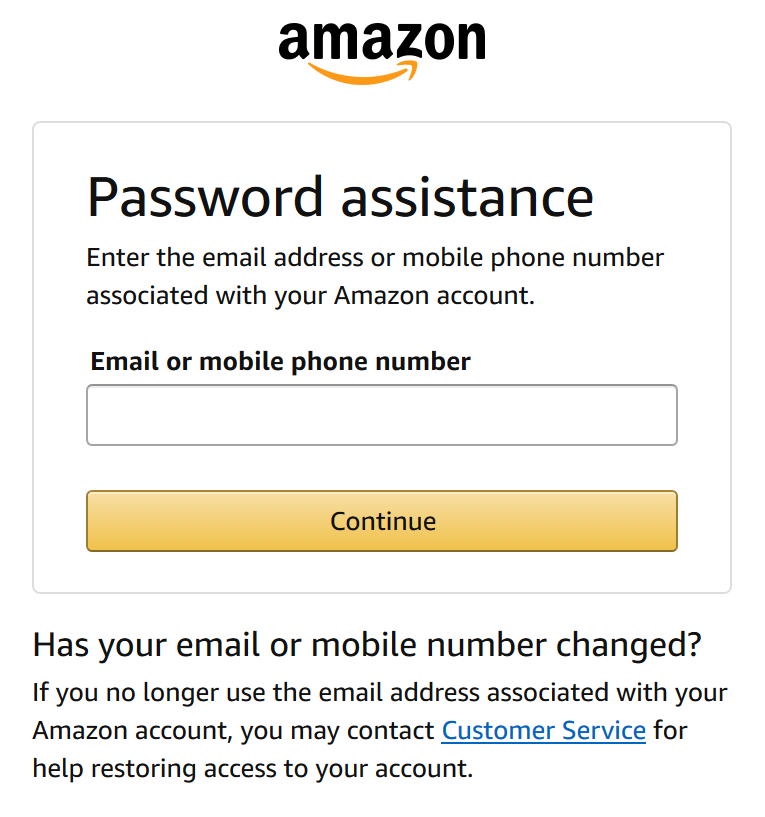The image displays an Amazon website page dedicated to password assistance. At the top center of the page, the Amazon logo is prominently featured in lowercase black letters, accompanied by an orange arrow forming an upward curve like a smile beneath it. 

A thin line outlines a rectangular section in the middle of the page. Inside this rectangle, on a white background, the title "Password assistance" is showcased in large, bold black letters with the 'P' capitalized. 

Below the title, instructions are provided in regular black print: "Enter the email address or mobile phone number associated with your Amazon account," with the 'A' in Amazon capitalized. Another bolded heading reads "Email or mobile phone number," with the 'E' capitalized.

Beneath this heading, there is an input field for entering the email address or mobile phone number. Following this input field is a yellow button of the same size that reads "Continue" in black print.

Outside of the square, towards the bottom, additional text offers further assistance: "Has your email or mobile number changed? If you no longer use the email address associated with your Amazon account you may contact customer service for help restoring access to your account."